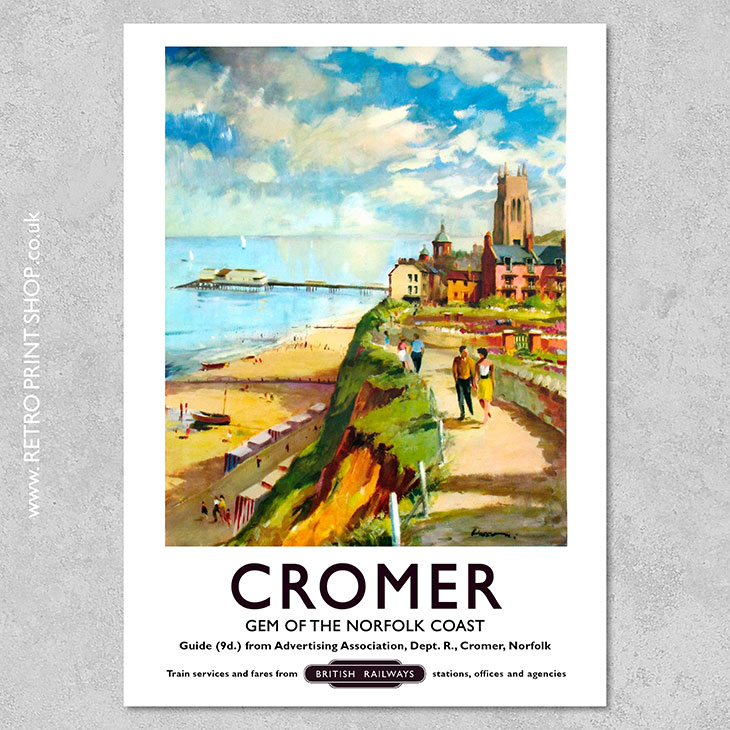This poster features a vibrant and picturesque scene capturing the essence of Cromer, a gem of the Norfolk Coast. The central artwork showcases a bright blue sky adorned with fluffy white clouds, reflecting on the glassy water below. In the foreground, there's a hill covered with lush, vibrant green grass. Scattered across the landscape are various buildings, mainly in light pink, orange, and beige hues, which add a charming touch to the scenery. A sandy yellow sandbank adds a warm tone to the picture.

Prominently, a couple walks toward the viewer along a quaint sidewalk, the man on the left and a woman on the right, who is wearing a striking yellow skirt. Around them, other individuals can be seen walking as well. At the bottom of the image, in bold black capital letters, is the text "CROMER, GEM OF THE NORFOLK COAST." Below, it reads, "Guide 9d from Advertising Association, Dept. R, Cromer, Norfolk. Train services and fares from British Railways stations, offices, and agencies," also in black text.

The poster itself is framed by a soft gray-beige background with a white border along the top and sides. Diagonally on the left side of the gray background, it reads www.retroprintshop.co.uk in white font, indicating where these retro prints can be obtained.